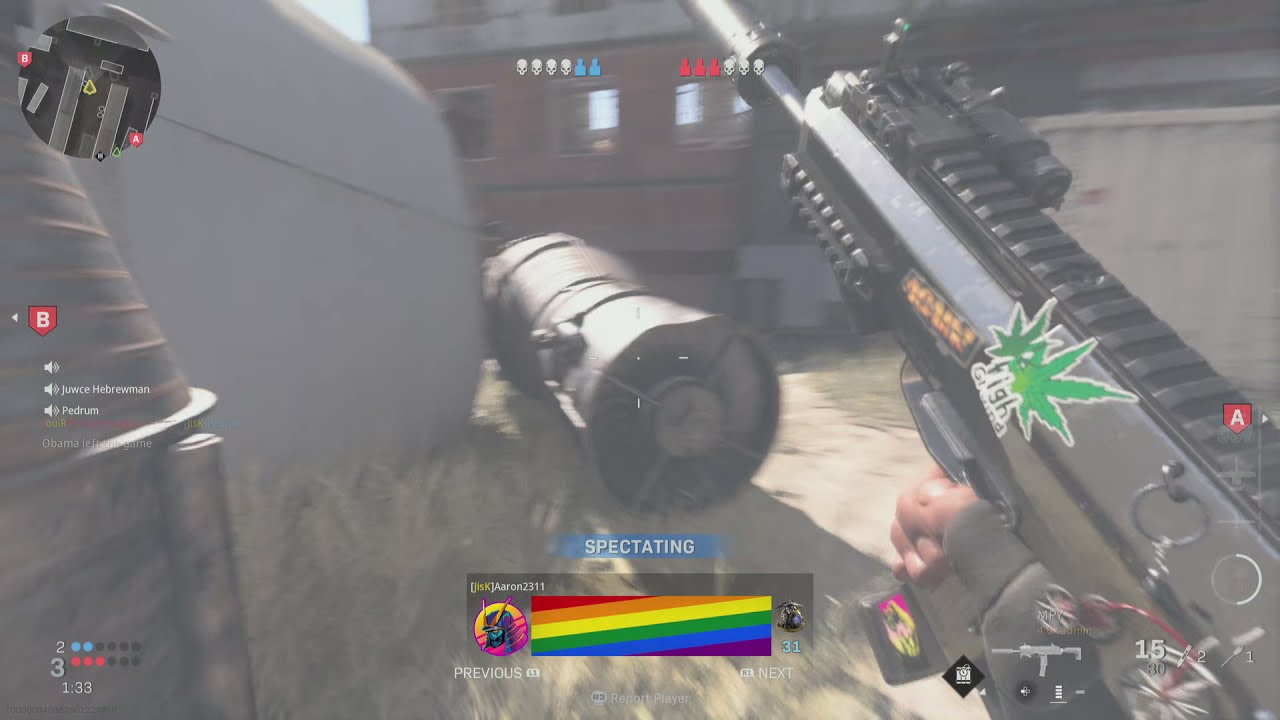This image is a detailed screenshot from a first-person shooter video game, depicting an intense warzone scene under daylight. The image captures a variety of objects and interface elements. Prominently, a player's gun, resembling an automatic Uzi, extends from the lower right towards the upper center. The foreground features a blue banner with white text that reads "spectating," indicating that the player is observing after being eliminated. Below this banner are controls for navigating different players, labeled "previous" and "next."

On the top left, there’s a circular radar, presumably for navigation or detecting enemies. Towards the bottom, the game interface displays a score and a timer for the current round. A multicolored horizontal bar (red, orange, yellow, green, blue, and purple) appears in the lower section of the screen. To the left of the gun, a large tubular structure, possibly a fuel container or a misidentified submarine-like object, dominates the scene. Further back, a toppled tower and a multi-story brick building with windows can be seen.

The color palette is diverse, featuring shades of black, red, blue, along with various other colors, creating a chaotic yet vibrant battlefield atmosphere. In the lower-left corner, a board displays blue and red dots, possibly representing team scores or player statuses, adding to the detailed gaming interface.